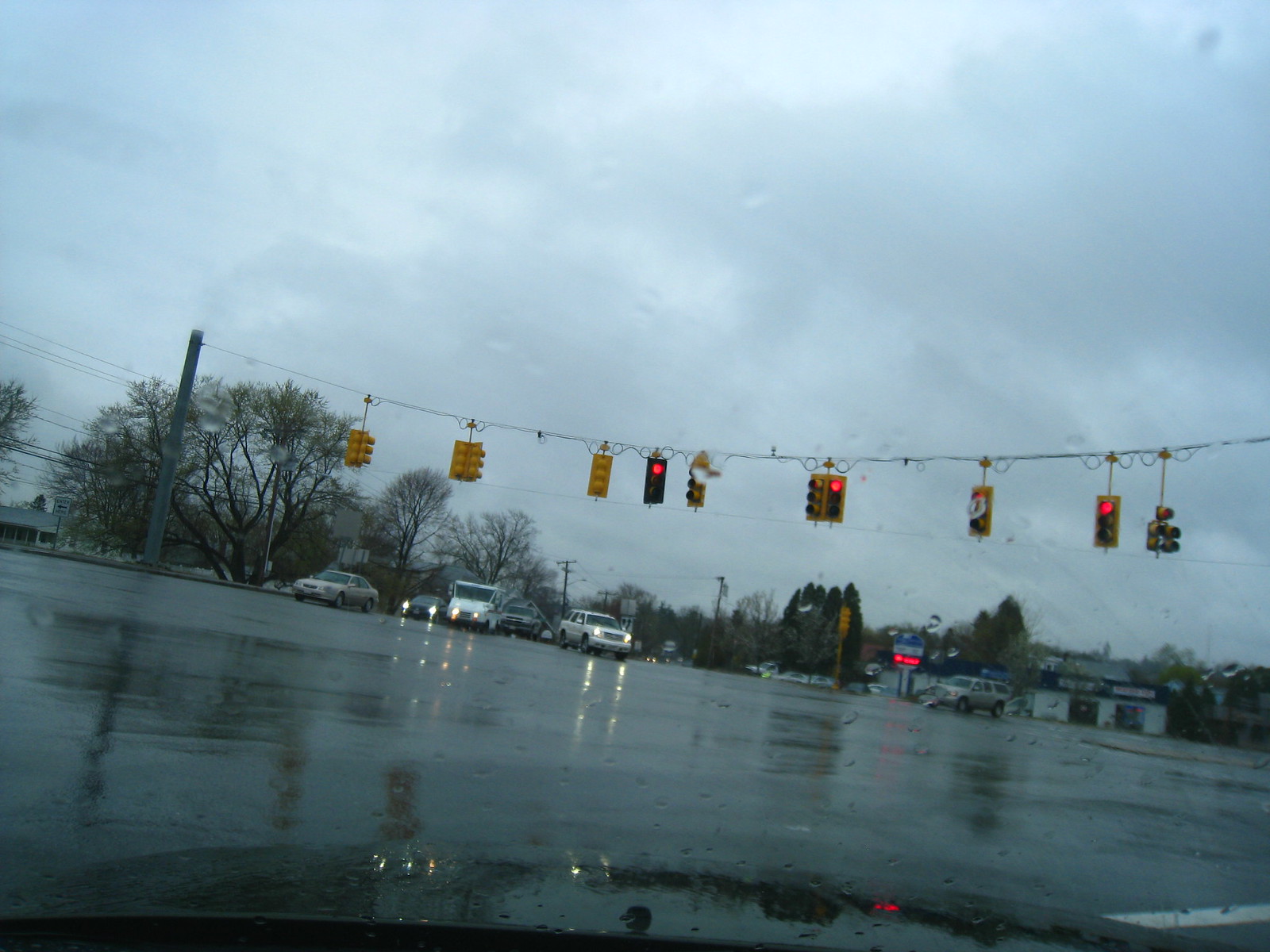The photo captures a rainy intersection scene from the perspective of someone inside a car, as evidenced by the visible car hood at the bottom of the image and water splashes on the windshield. The gray, overcast sky forms a somber backdrop, while the wet asphalt reflects the lights and surroundings, confirming the rainy weather. In the foreground, a series of traffic lights line up, all showing red signals. A mix of vehicles, including a mail truck, a silver SUV, a silver sedan, and a gray SUV, populate the intersection, some poised to turn. Distant, leafless trees and a building that resembles a restaurant with a blue roof and an accompanying sign mark the background. The scene exudes a typical gloomy day at a busy crossroad.